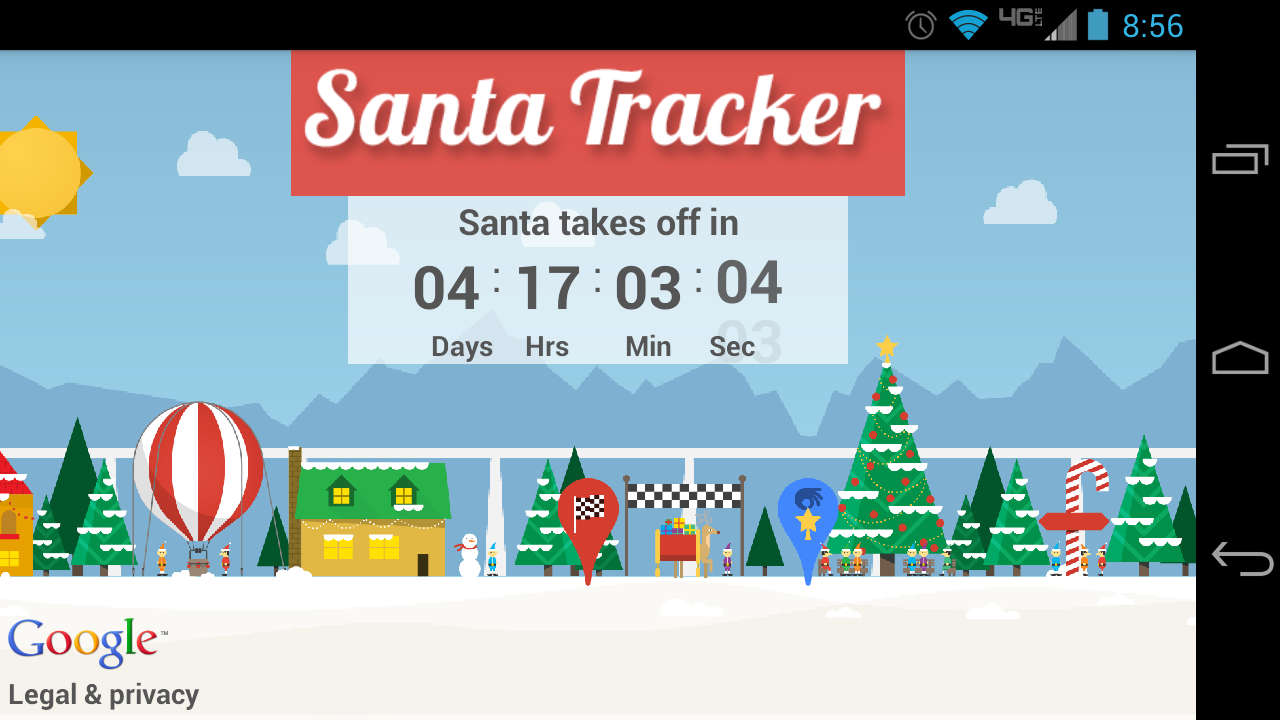Screenshot of a mobile phone in portrait mode displaying a festive website. At the top, the black status bar features several icons: an alarm clock, full Wi-Fi signal in blue, 4G in gray font, one out of five mobile signal bars, a blue battery icon, and the time, 8:56. On the right side, typical navigation icons for home, minimize, and back are lined up in a black bar.

The main content showcases a cheerful, illustrated scene of a snowy town under a blue sky with the sun and clouds. Mountains are visible in the background, while the foreground features snow-covered ground, a small house, a snowman, and decorated Christmas trees with presents. At the very top, a red rectangle with white font reads "Santa Tracker." Below this, a translucent white square displays a countdown timer in black font, stating "Santa takes off in 04:17:03:04."